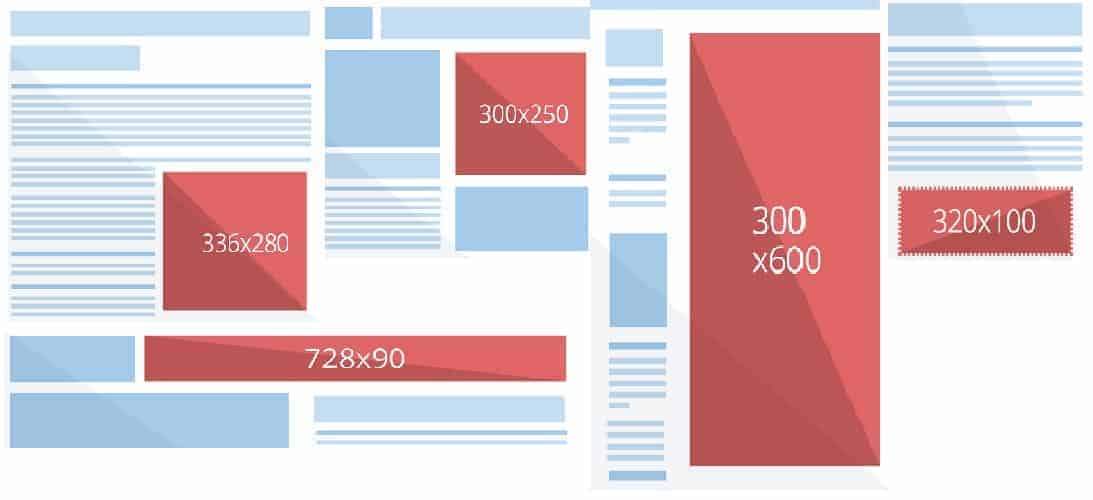This image features a variety of colored shapes and text, each marked with specific dimensions and colors. On the left side, blue lines or a bar are visible. To the right, a square identified as "light red" is present. In the bottom left corner, there's a darker colored area. Adjacent to the right side, text reading "336628" can be seen.

At the bottom of the image, a rectangle labeled "728x90" is displayed. Towards the top, another rectangle marked "300x250" is shown, characterized by its blue color. The top right corner features another blue geometric shape or area with lines.

On the far left, a vertical column with the dimension "300x600" is visible. This column, or rectangular shape, stands out amidst others. Additionally, within this array of shapes, a white rectangle labeled "320x100" can be found, positioned among what appears to be some dark shadows in the background.

The overall background of the image is white, providing contrast and clarity to the various colored elements and dimensions mentioned.